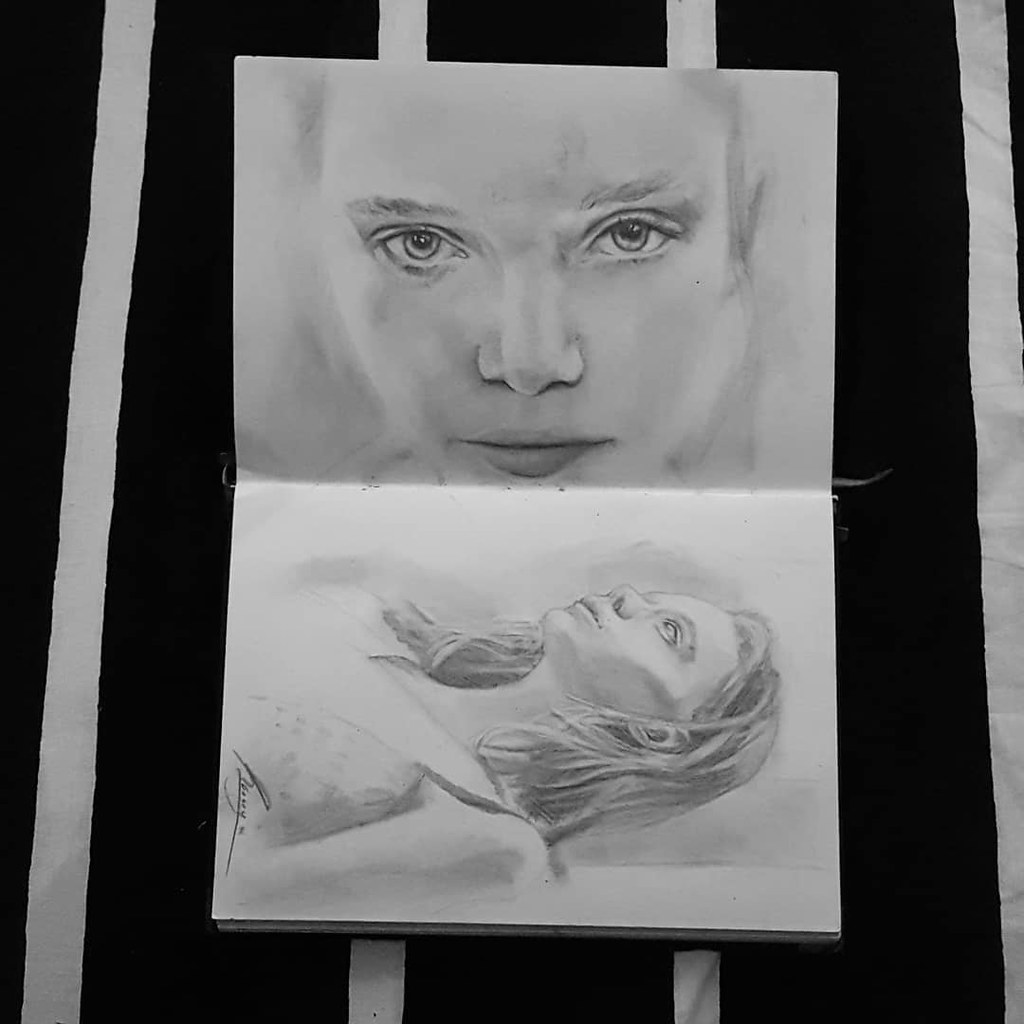The image showcases a black-and-white pencil sketch drawn on a white piece of paper that is folded in half. The artwork features two distinct portraits of a young Caucasian female. 

The top half of the image is a close-up of the girl's face, capturing her delicate features in painstaking detail. Her eyes are prominently drawn, with defined eyebrows above them. The sketch includes her nose and a neutral expression on her lips. Although she has no visible hair in this section, there is a subtle indication of a right ear.

In contrast, the bottom half of the image provides a profile view of the same teenager, emphasizing her right side. This portrait includes her shoulder-length hair that drapes gently, complementing her slender neck and part of her torso. She is depicted wearing a light-colored dress, though the exact hue remains indeterminate due to the monochromatic nature of the drawing. The profile captures her delicate frame and the youthful grace of a slender, young female.